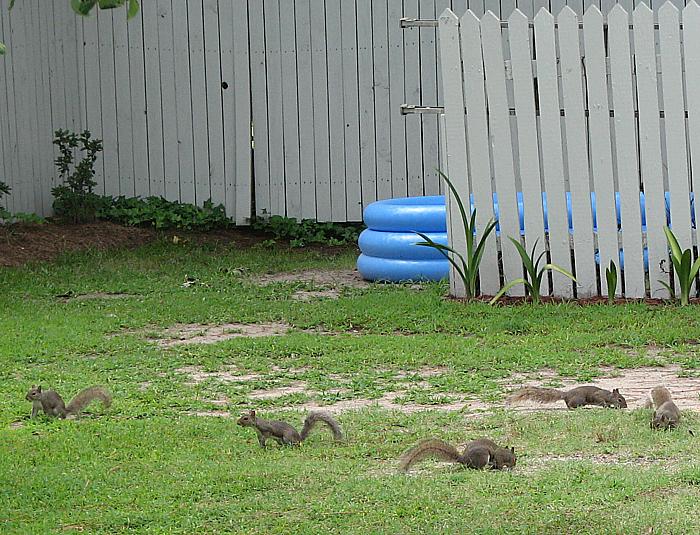In the photograph, five squirrels, varying in shades of dark gray and brown, are scattered across a patchy lawn that exhibits both green grass and exposed dirt. The squirrels are engaged in different activities; three of them are foraging for food with their heads down, while the other two appear alert, standing with their tails upright. The yard is enclosed by a tall, white picket fence which has a gate that looks permanently open and displays metal hinges. Beyond the squirrels, there is a blue inflatable pool with three concentric rings, partially obscured by an additional standalone section of the white picket fencing. The pool area is flanked by an assortment of plants and flowers, with ivy growing along parts of the perimeter fence. To the left of the image, there is a berm with green plantings and the upper left corner shows a few leaves, likely from a nearby tree.